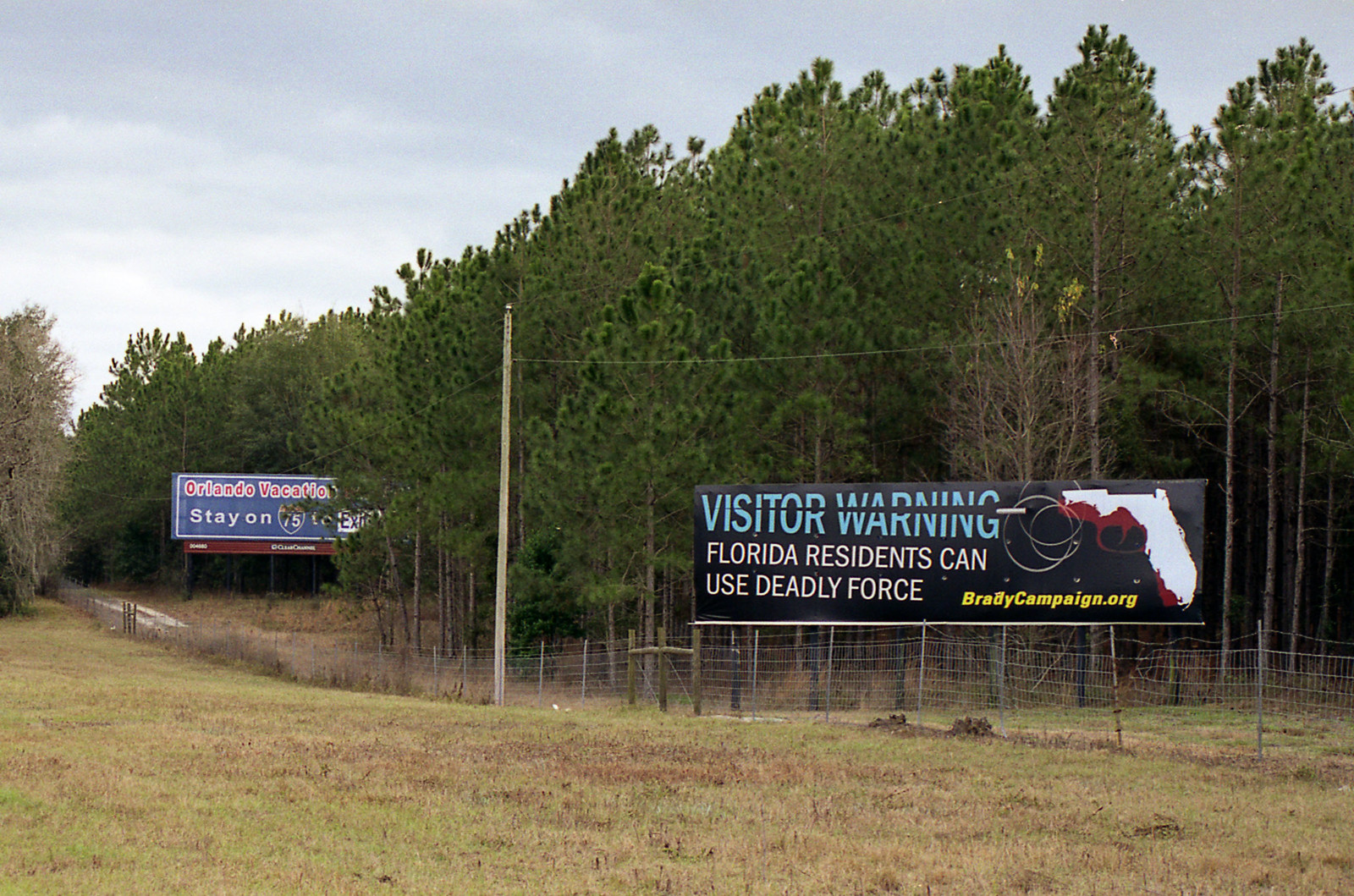This outdoor photograph captures a serene grass field fenced off with a simple wire barrier. Adjacent to the fence stretches a narrow dirt path, likely used for biking or hiking. Beyond the trail lies a dense forest of towering trees with thin trunks, their green canopies rustling in the gentle breeze. Two prominent signs catch the eye: a large billboard-style warning sign advising visitors of Florida residents' right to use deadly force, accompanied by a gun illustration, and another sign directing travelers toward Orlando vacations with the text "Stay on 75."